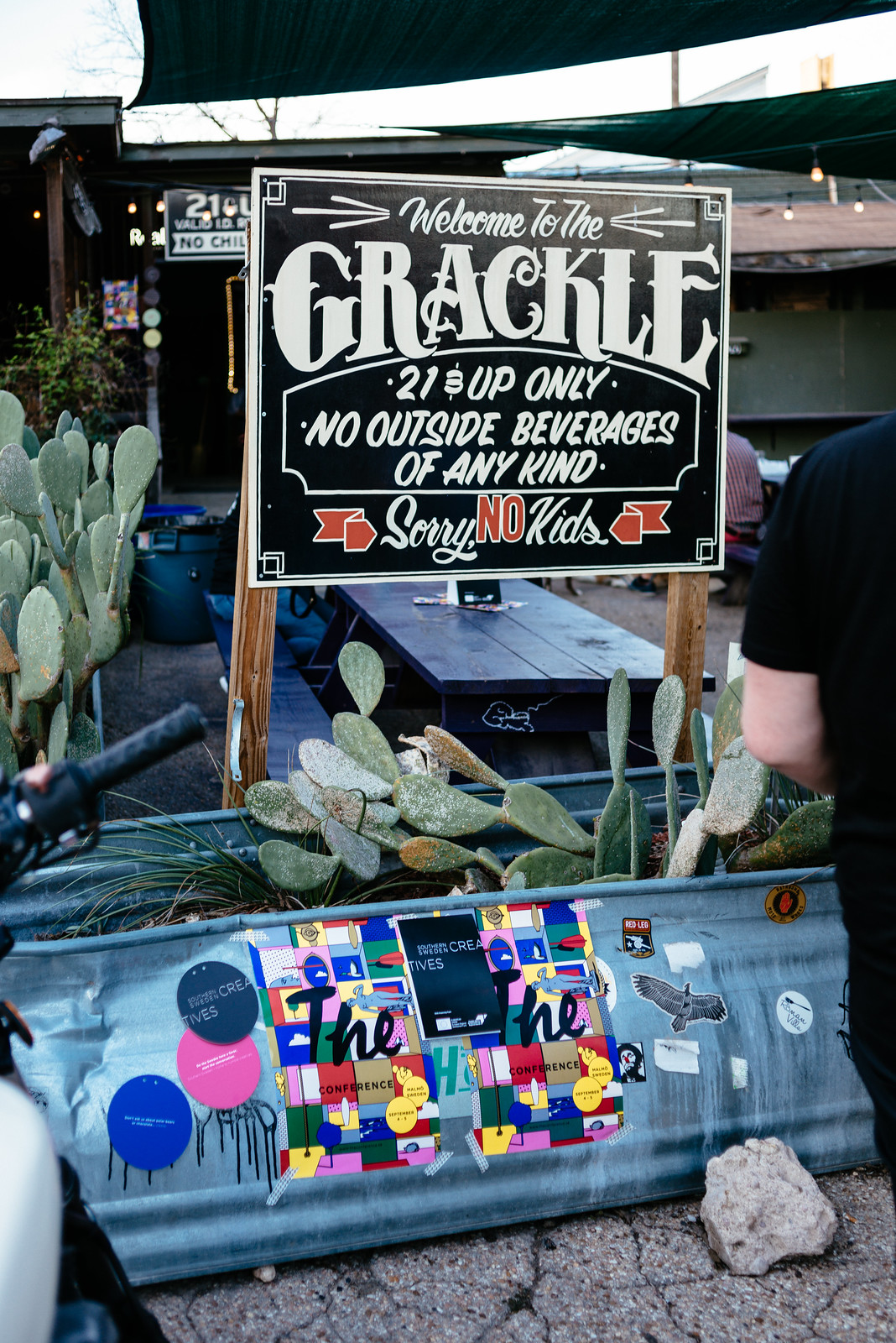In the image, there's a bustling outdoor bar scene set in the middle of the day, with a worn concrete surface at the bottom showing visible cracks and scattered rocks. At the center, a prominent sign reads: "Welcome to Grackle, 21 and up only, no outside beverages of any kind, sorry, no kids," written in white text. Surrounding the sign are artistic decorations, including various stickers and colorful shapes such as circles in blue, pink, and gray. In the background, to the left and right of the sign, there are tables and chairs, with people casually mingling. One noticeable figure is a man in a black shirt and shorts. Cactus plants are growing nearby, adding to the rustic ambiance. Behind everything, a blue aluminum wall forms the backdrop, adorned with eclectic and vibrant designs. The scene captures a lively, artistic atmosphere typical of a trendy bar or restaurant setting.